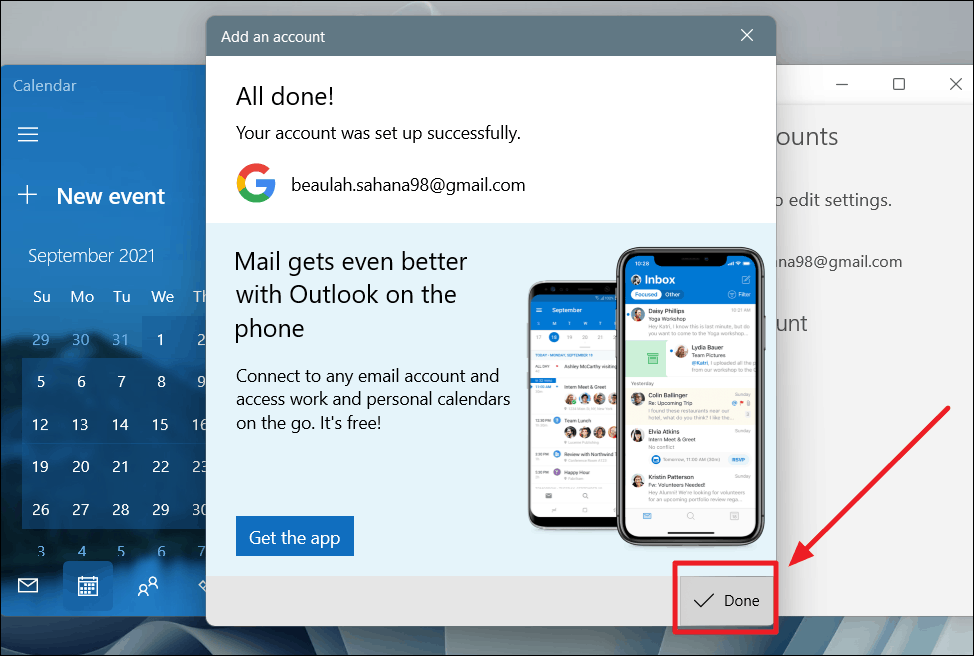The screenshot showcases multiple overlapping menus on a Windows desktop. In the background, partially visible on the left, is a blue and light blue calendar for September 2021, with white lettering, though it is cut off halfway. Dominating the foreground is a prominent window titled "Add an Account," indicating successful setup for the email address "Beluha at Sahana 98 at gmail.com." This window features a white or gray bar at the top with a small 'X' for closing it.

The message in this window reads, "All done. Your account was set up successfully," followed by promotional content encouraging the use of Outlook on mobile devices to access work and personal calendars on the go. Below this, there is a graphic of a couple of phones and a blue button labeled "Get the app" in white lettering. Adjacent to this, a black check mark and a button with "Done" are located at the bottom right, enclosed in a red square with a red arrow pointing to it.

Behind the primary window, on the right side, there's another obscured menu, likely an account settings menu, partially visible with some text and the familiar minimize, maximize, and close options at the top. The background of the desktop reveals part of a Windows-themed design at the bottom, confirming the operating system.

Overall, this image captures the process of someone configuring their Gmail account on a Windows PC.